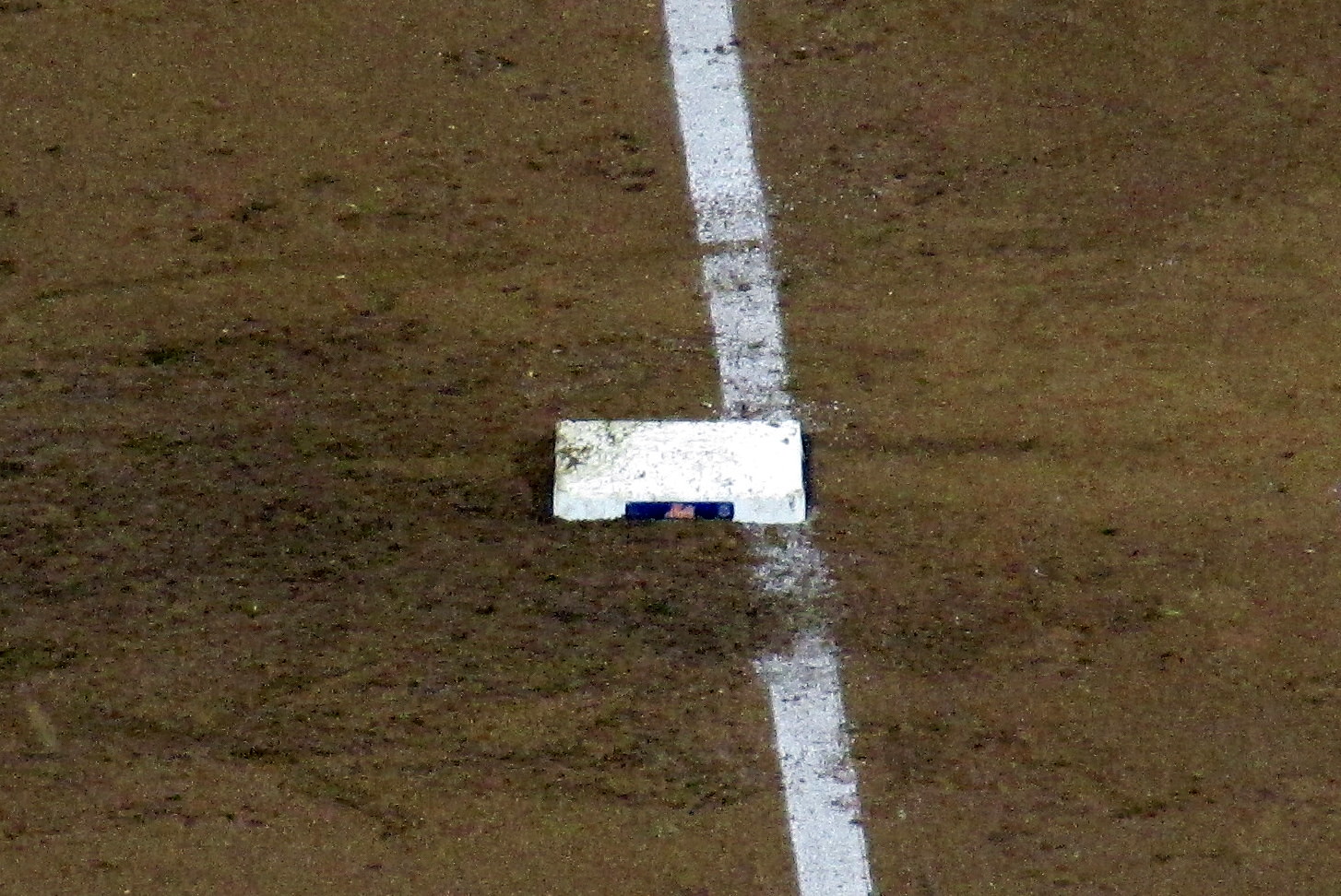The photograph captures a baseball base situated on a brown, muddy ground. A narrow white chalk line extends diagonally from top left to bottom right, with parts of the chalk line broken up by players' foot traffic. The base, appearing dirty with some brown soil, is positioned at the center of the image and is a key focal point. The white square base, resembling a fabric tile, is embedded into the ground with the chalk line running just along its edge. There seem to be markings or a logo, possibly with an orange-ish font on a blue background, that might indicate a baseball team like the Mets, though the details are not entirely clear. The base is part of the runner's track, suggesting the setting is a baseball field, where players tag this base as they run.